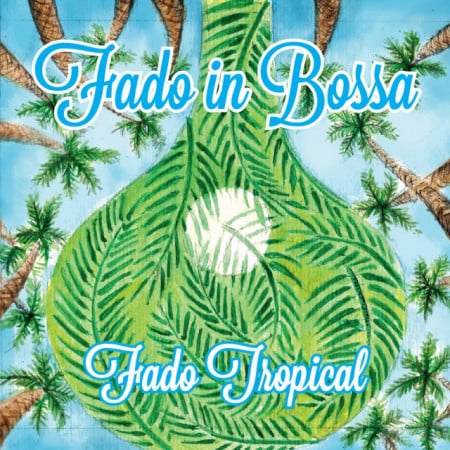The image is a detailed drawing with a tropical theme, titled "Fado in Baza." The title is prominently printed in blue letters at the top, each letter outlined with white. At the center of the image, there is a bell-shaped structure reminiscent of a green vase, adorned with intricate, dark green leaf patterns. In the midst of this central green shape is a conspicuous white circle, partially veiled by the leaves. The backdrop of the drawing reveals a vibrant blue sky peeking through sporadic white clouds, heightening the tropical ambiance. Flanking both sides of the image are numerous tall palm trees, each with brown trunks and lush green fronds. Towards the bottom of the illustration, the text "Fado Tropical" is displayed in white letters bordered by blue, which stands out against the verdant scene. This visually stimulating composition conveys a sense of being immersed in a verdant, sun-drenched tropical paradise.